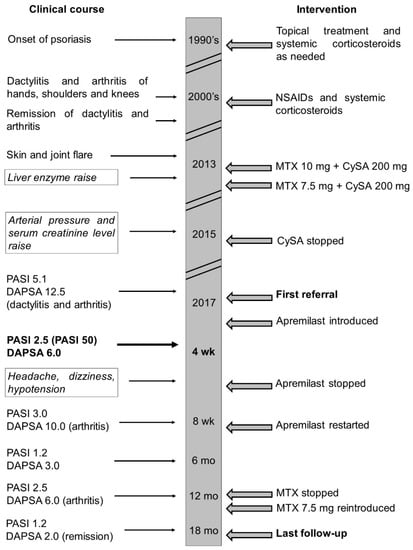The image is a detailed time chart mapping the clinical course of a patient with psoriasis and corresponding medical interventions over multiple years. The chart consists of three columns: the left column titled "Clinical Course," the middle column as a gray vertical bar delineating different time periods, and the right column titled "Intervention." Starting from the top, the gray bar is marked with time periods including the 1990s, 2000s, 2013, 2015, 2017, followed by 4-week, 8-week, 6-month, 12-month, and 18-month intervals. 

Under "Clinical Course," the chart contains sequential events: onset of psoriasis, dactylitis and arthritis affecting hands, shoulders, and knees, remission of dactylitis and arthritis, a skin and joint flare, a rise in liver enzyme levels, an increase in arterial pressure and serum creatine levels, PASI and DAPSA scores, headaches, dizziness, hypotension, and recurring arthritis. These clinical events are marked on the timeline with arrows pointing to the specific time periods they occurred.

In the "Intervention" column, corresponding treatments are listed, beginning with "topical treatment and systemic corticosteroids as needed" during the 1990s, and continue parallel to the progression of clinical symptoms on the timeline. This comprehensive layout provides a detailed overview of the patient's medical history, symptoms, and treatments over time.